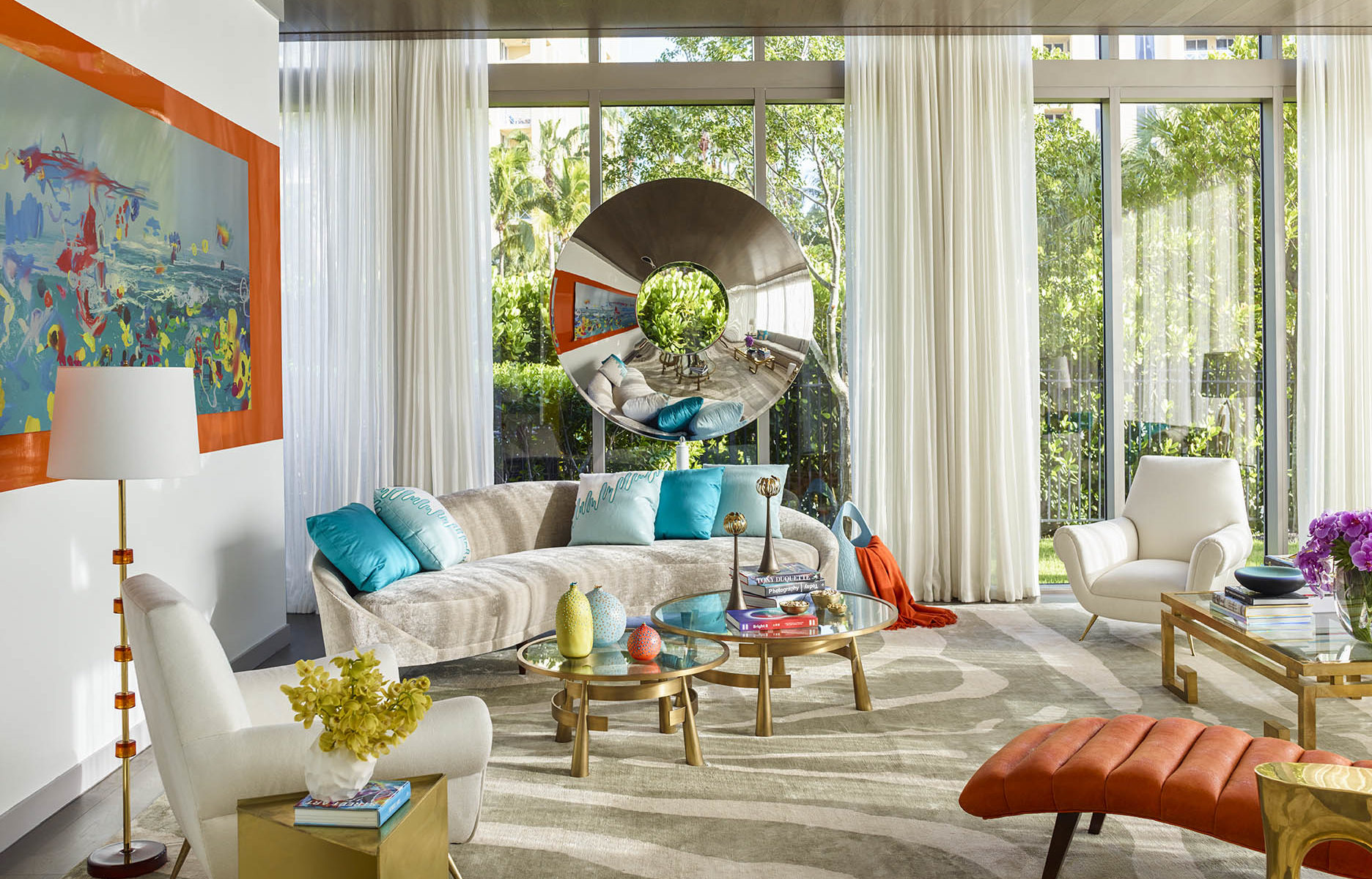The image depicts an elegantly decorated, expansive living room bathed in natural sunlight through large glass windows adorned with floor-to-ceiling white drapes, revealing a view of lush green trees outside. The high-ceilinged space features a meticulously maintained cream and tan carpet with intricate designs. The furniture predominantly includes a chic white and cream couch accented with five blue pillows, and a distinctive curved orange lounger in one corner. A matching rust-colored chaise adds a splash of warmth. 

Two round wooden coffee tables accompany a contemporary brass and glass coffee table, which is adorned with vibrant purple flowers, an assortment of books, and a striking blue decorative bowl. Additional round coffee tables are adorned with various tasteful decor items. A chic silver circular chair is also visible in the distance. 

Artistic touches include a large ornate painting on one wall and a unique abstract artwork, offering colorful visuals that may resemble either flowers or fish. A visually intriguing round bullseye mirror with a donut-like cutout offers a reflective perspective of the room, enhancing the overall aesthetic. Tall, slender floor lamps contribute to the modern, clean, and somewhat sterile ambiance of the room, which is accentuated by the pristine, cream-colored carpet. The space is undeniably luxurious, emphasizing both contemporary elegance and meticulous attention to detail.